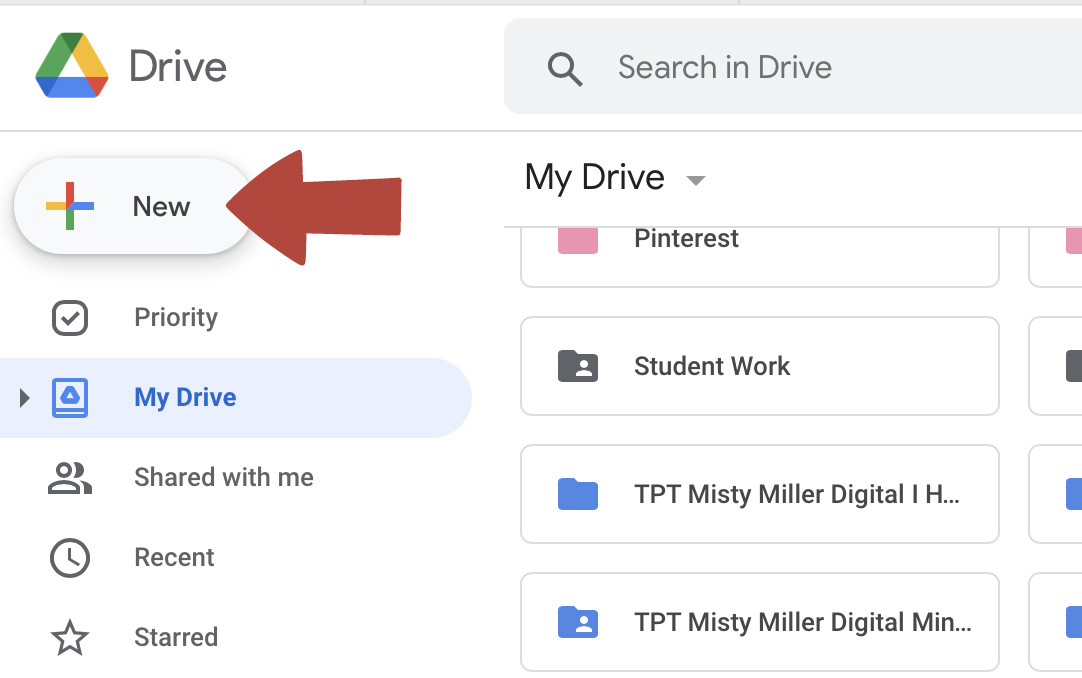The image displays a Google Drive screen interface. Dominating the top left corner is the recognizable Google Drive logo, painted in a triangular motif with green, yellow, blue, and red colors. Adjacent to the logo, a search bar labeled "Search and Drive" offers functionality to find files within the drive.

Underneath the search bar, the "My Drive" section is highlighted prominently. Several folders and buttons are visible, including "Pinterest," "Student Work," "TPT," "Misty Miller Digital," and "IH." A repeat of "TPT" and "Misty Miller Digital" folders, along with a folder labeled "MIN," are also present in this primary viewing area.

On the left sidebar, there are multiple navigational options. At the top of this sidebar, a "New" button allows users to create new files or folders. Below this, the "Priority" section is featured, followed by "My Drive." Further down, a "Shared With Me" option is depicted with an icon illustrating two simplified human figures. Other sections include "Recent," and "Starred," the latter indicated by an accompanying star symbol.

This detailed layout portrays the organizational structure and various interactive elements available to a Google Drive user, highlighting the accessible tools and files within their digital workspace.